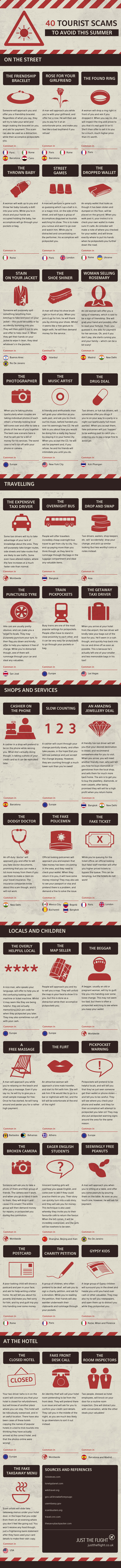A vertically narrow, rectangular image outlines a detailed list titled "40 Tourist Scams". The list is meticulously sectioned into three columns, each comprising multiple sections. These sections are distinguished by horizontal black banners, making the organization of the content easier to identify. Though the text within each section is challenging to read due to the image's limited clarity, the overarching theme is clear: it details various scams that unsuspecting tourists might encounter. The background of the image is an off-white shade, providing a neutral canvas for the information. Black text fills each description box, accompanied by small, red-printed images whose specific details are difficult to discern. The overall composition suggests a comprehensive guide aimed at educating and protecting travelers from common pitfalls during their journeys.